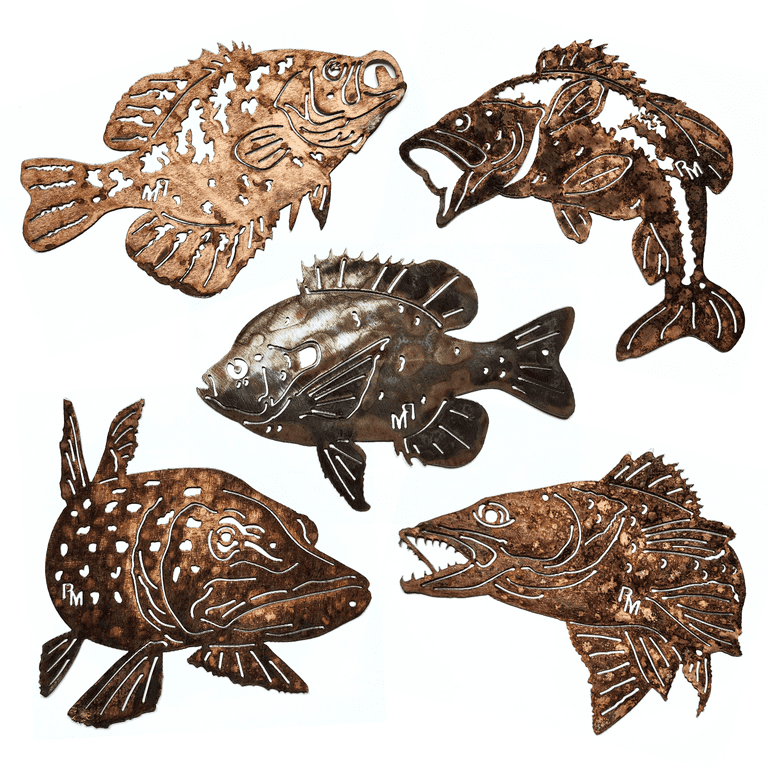This image showcases five intricately detailed metal fish sculptures, each varying in shape and size, on a plain white background. The fish appear to be crafted from a copper or brassy gold material, giving them a metallic, dark brown to light brown appearance, with one in the center being notably darker, nearly black. Each fish sculpture exhibits a unique pose, with some having open mouths and sharp teeth, indicative of species like a piranha. The top left fish, the lightest in color, faces diagonally upwards to the right with its mouth open, featuring prominent fins and a long tail. The top right fish, darker in color, also has an open mouth, a distinct top fin, and detailed etchings. In the center, a dark brown fish with a slightly open mouth has three visible fins, one large at the top and two at the bottom, along with a predominantly black tail. The bottom left fish, a mix of brown and light brown, has a closed mouth, contrasting with the bottom right fish which is slightly lighter, mouth open showcasing sharp teeth. Each sculpture is meticulously laser-cut, with detailed eyes, tails, fins, gills, and the monogram "P.M." engraved near the belly or tail, adding to their artistic and decorative appeal.